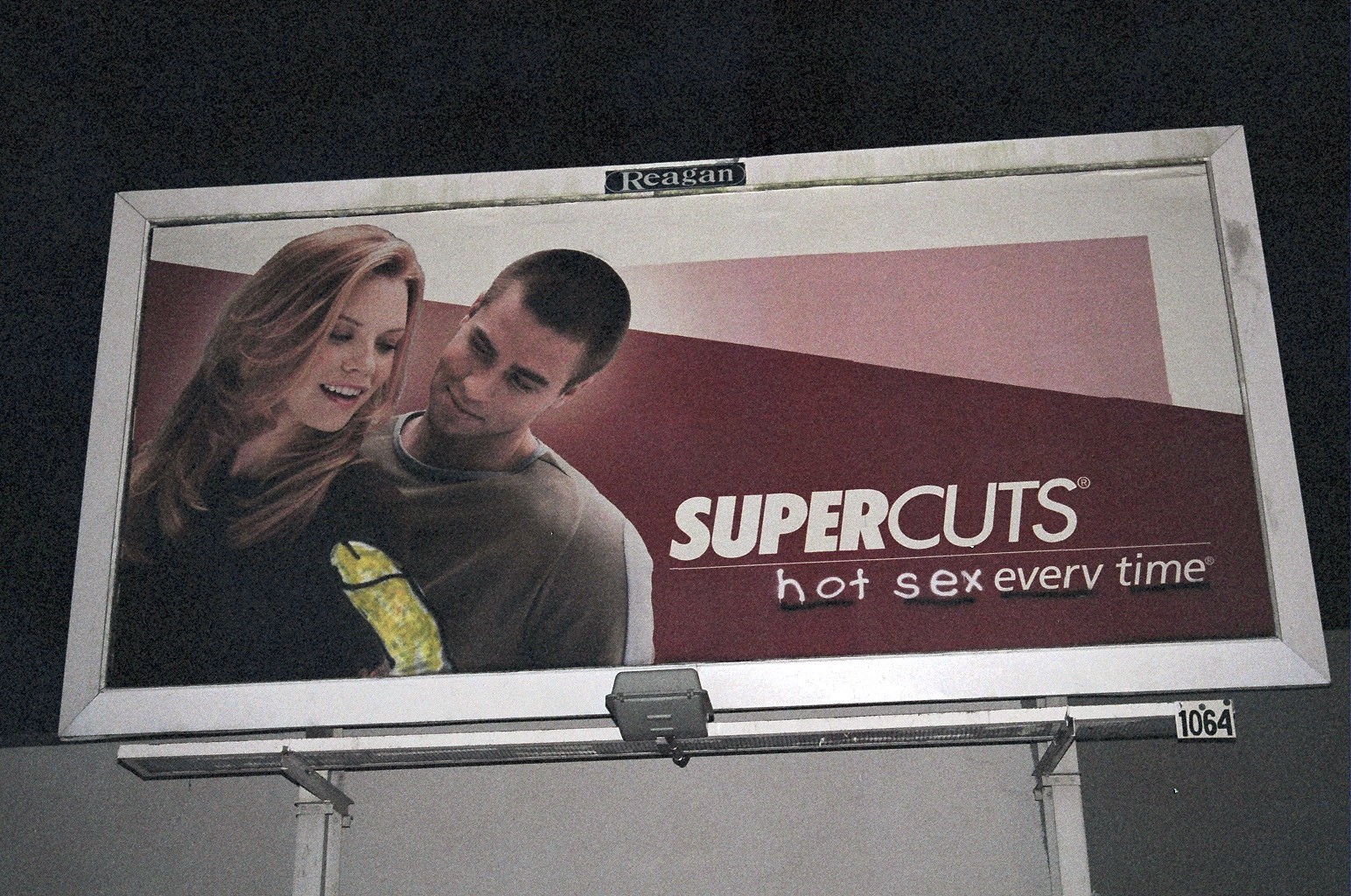The image features a nighttime photograph of a billboard framed in white with the brand name "Regan" visible along the perimeter. The billboard, illuminated by a light at the bottom, displays an advertisement for Supercuts. The background transitions from red to pink and then to white, resembling a cut pattern in line with the Supercuts theme. The ad showcases a young, attractive man and woman who appear to be quite happy, looking and smiling at each other in close proximity. Originally, the billboard reads "Supercuts, every time," but someone has graffitied the words "hot sex," making it read humorously as "Supercuts, hot sex, every time." The photograph captures only the billboard against the darkness of the night sky, emphasizing its illuminated presence.